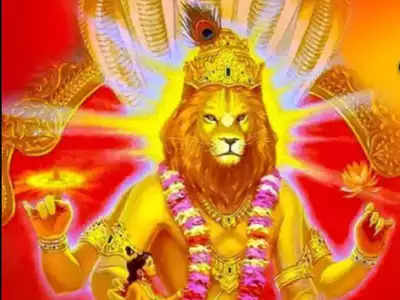This vibrant and intricate artwork depicts a multi-armed being resembling a fusion of human and lion, symbolizing cultural motifs that hint at Indian influence. The central figure, with four arms, has the head of a lion, crowned with an ornate gold crown adorned with a peacock feather. Its cascading mane adds to its majestic presence. The figure's neck is draped with a colorful lei made of red, yellow, and pink flowers, complemented by a gold chain necklace featuring a prominent square medallion. The creature's hands hold various items: one hand points upward encircled by a golden ring, while another holds a flower. The other two hands rest by its sides, each arm festooned with bracelets or arm cuffs. 

The backdrop is a radiant red, accentuated by a golden archway and a sunburst effect of radiating beams behind the head, symbolizing divinity or enlightenment. Below and slightly off-center, a small woman with dark hair and a crown gazes up at the creature, possibly indicating reverence or worship. She adds an element of human interaction to this divine tableau. The throne-like setting and the detailed ornamental work emphasize the majestic and sacred nature of the figure, making this piece both beautifully artistic and deeply symbolic.